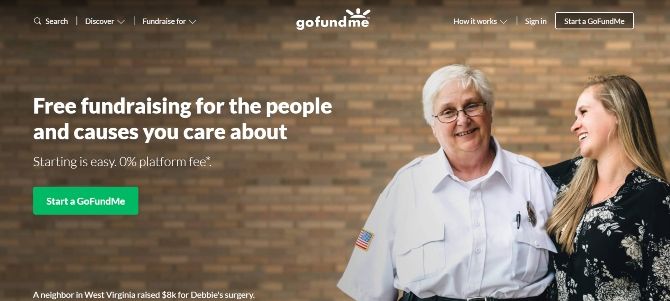This image is from a GoFundMe page, featuring two women standing in front of a brick wall on the right side. The older woman, clad in a white uniform adorned with an American flag on the right sleeve, has white hair and glasses, and she is facing the camera with a warm smile. Beside her, to the right, is a younger woman with long blonde hair, wearing a blue shirt with white floral patterns, looking at the older woman and smiling.

The top left of the image displays the text "Search, Discover, Fun For," while the center top reads "GoFundMe." On the top right, the text reads: "How It Works," "Sign In," and there is a "Start a GoFundMe" button. Positioned on the left, towards the center, the text proclaims, "Free Fundraising for People and Causes that You Care About," followed by "Starting is Easy, 0% platform fee." Below this, a green button with white letters reads, "Start a GoFundMe." At the bottom left corner, the image highlights, "A neighbor in West Virginia raised $8,000 for Debbie's surgery."